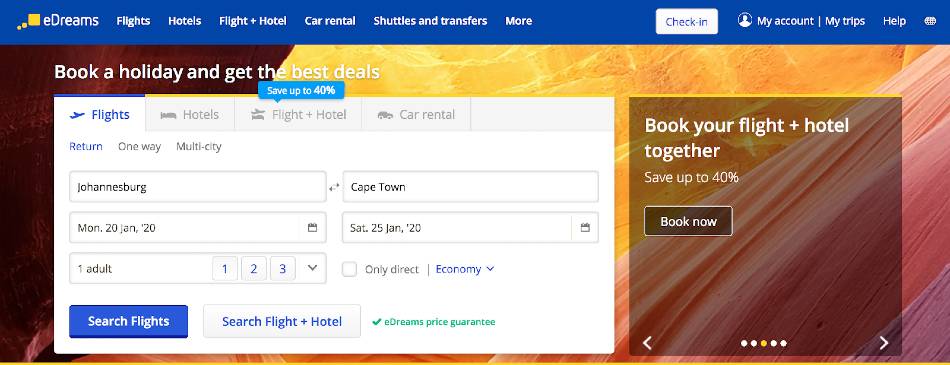The image shows a screenshot of the eDreams website homepage. The header, approximately an inch tall, spans the full width of the page in a vibrant blue color. Situated in the top left corner, there is a red square icon flanked by two smaller yellow squares to its lower left. Right beside this icon, the brand name "eDreams" is prominently displayed in white text.

Just below the brand name, there's a navigation menu featuring clickable tabs: "Flights," "Hotels," "Flight + Hotel," "Car Rental," "Shuttles & Transfers." Separately, there's a white tab with "Check In" written in blue on it. Further to the right are personalization options, including a small profile icon next to the text "My Account," followed by a dividing slash, and then "My Trips," and "Help." In the top right corner, a small circular icon is visible.

The section below the blue header features a textured burgundy background, which transitions diagonally left to right into yellow, followed by pink, and ultimately purple in the rightmost corner. On the left side of this section, in bold white letters, it says "Book a holiday and get the best deals." Directly below the word "best," there is a small blue rectangle with "Save up to $40" in white within it.

Further down, there is a search box interface with tabs for booking: "Flights" in blue, "Hotels," "Flight + Hotel," and "Car Rental" in gray. Below these tabs, fields for entering travel details such as address and date are provided. At the bottom left of this segment, there is a blue button with "Search Flights" in white text. To its right, a semi-transparent pop-up with a yellow outline contains a white message stating "Book your flight + hotel together." Below this, in yellow text, it says "Save up to 40%," accompanied by a black button marked "Book Now" in white letters.